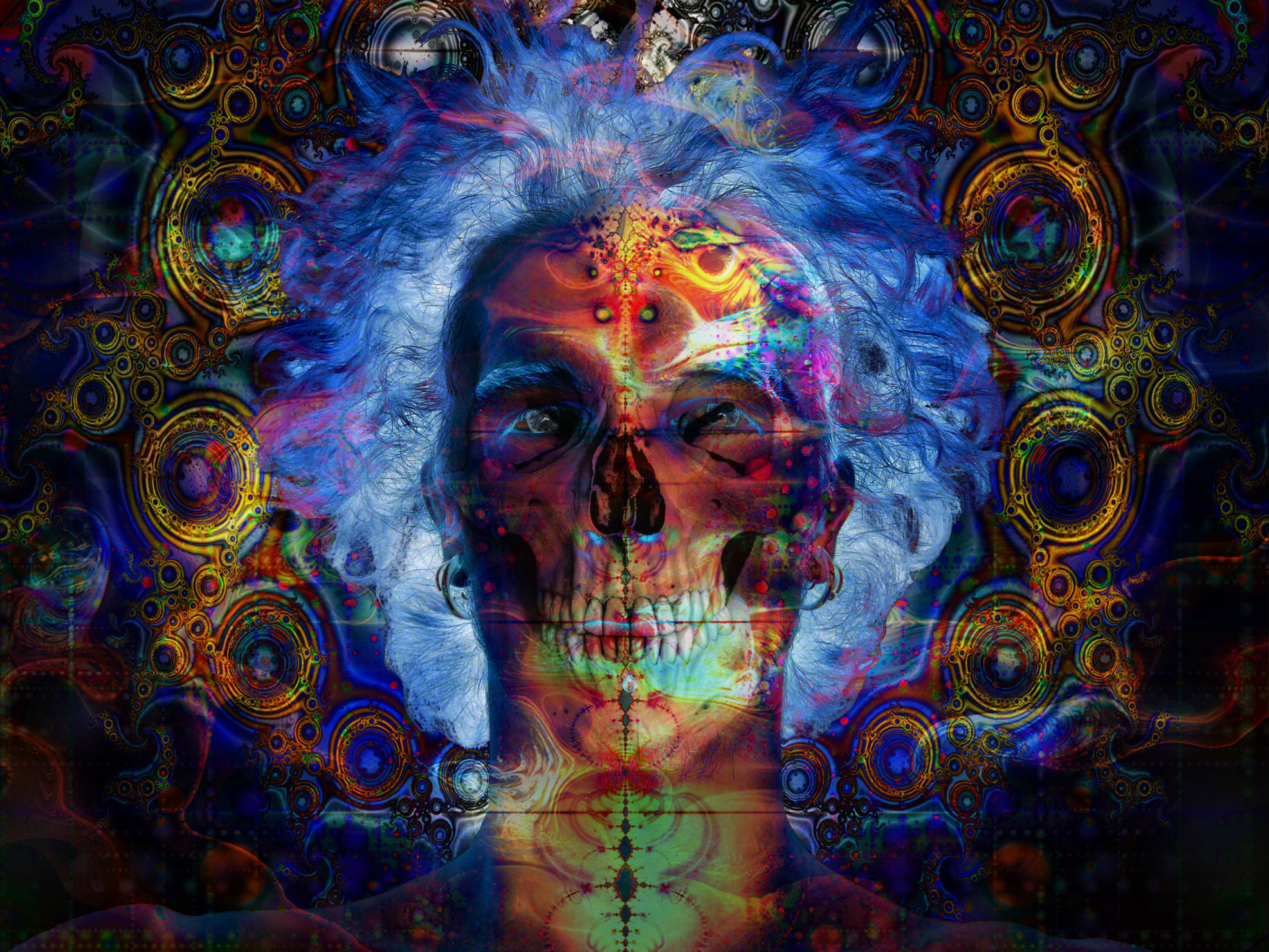This vibrant and psychedelic digital painting centers on a hybrid human head and skull, revealing detailed anatomy from the shoulders up. The muscular shoulders transition into a more skeletal visage, with visible jawbones, rows of teeth, and a nose showing intricate bone structure. The hollow eyes reveal the elongated shapes, pupils, and colorful eyebrows, highlighted in hues of light blue, dark blue, and pink near the crow's feet. The piercing-adorned ears add a touch of surreal realism to the image. The neck displays bright, vibrant yellow rings interspersed with various shades of gray and red where the spine would be. The head is adorned with sky blue hair, wispy and flowing just below the shoulders, rendering a glowing effect with colors ranging from oranges, yellows, and greens to browns, as if illuminated by a bright white light at the back. Surrounding the central figure, a mosaic of dark and light blues, coupled with concentric yellow rings that appear almost quilt-like, extends outward. Enhancing this psychedelic aura, gold-tinged circles and blue-centered yellow rings create an intricate, evolving pattern, intensifying towards the edges of the painting.